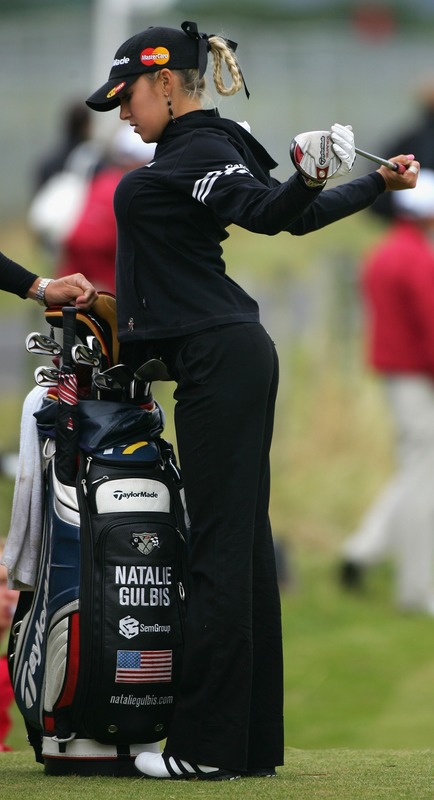In this photograph, Natalie Gulbis, a professional female golfer, is prominently featured in the center of the image. She is captured in a left profile view, looking down toward the ground and facing to the right. Natalie is in the midst of a stretch, holding a golf club behind her back with both hands. She is donning a coordinated black athletic outfit, consisting of long black pants, a black jacket with a white stripe, and a black cap emblazoned with the MasterCard logo. Her blonde hair is styled in a braid that loops up into her cap, and she wears a white glove on her left hand. Her footwear includes distinctive white and black saddle golf shoes. To her left, her personalized, colorfully decorated golf bag prominently displays her name, “Natalie Gulbis,” along with features such as the American flag and red, white, and blue accents. The bag also holds five golf clubs. A hand, belonging to an unseen individual, rests on top of the bag. The background is blurred, but it is clearly a sunny day as two indistinct figures clad in red and white attire walk past, further emphasizing the focus on Natalie.